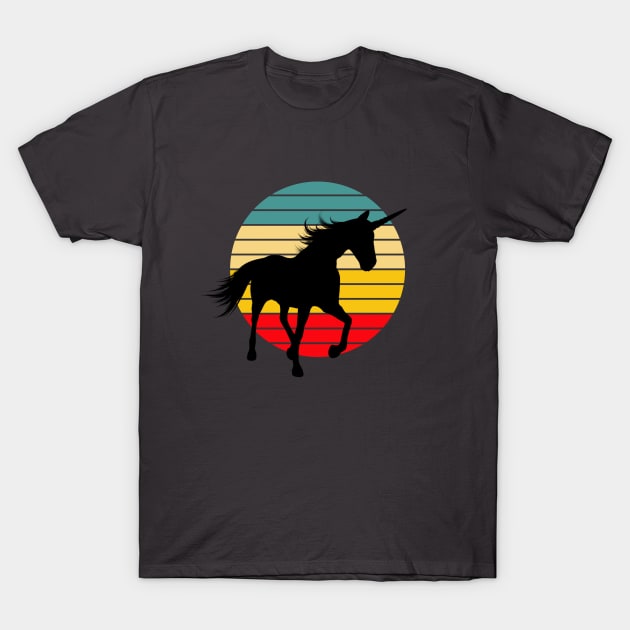The image features a black t-shirt as its primary subject. At the center of the t-shirt, a striking black unicorn stands majestically. Behind the unicorn, a vibrant circle formed by horizontal bars adds a dynamic backdrop. The circle comprises an array of bars starting with three in a teal green shade, followed by three beige-yellow bars, then transitioning into three bright yellow bars, and finishing with three red bars. This colorful arrangement of horizontal bars creates a captivating and contrasting ring behind the black unicorn, enhancing the overall appeal of the t-shirt design.